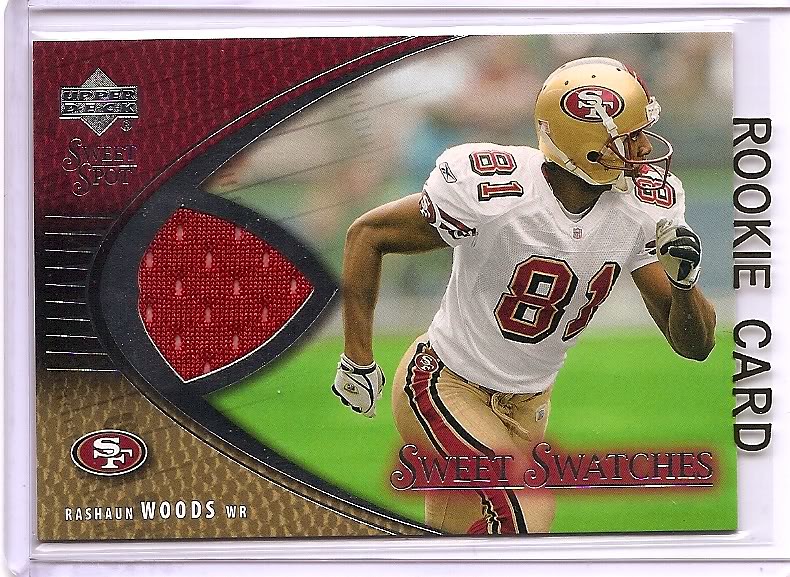This image features a detailed view of an NFL football card with a primary focus on San Francisco 49ers wide receiver Rashawn Woods. The card itself is predominantly in the team colors of red and gold and is bordered in white, suggesting it is in a protective sleeve. 

In the top left corner, the card showcases the silver "Upper Deck" logo with a diamond shape beneath it, overlaid by a rectangle and accompanied by a trademark "R" symbol. Below this, in equally silver lettering, the words "Sweet Spot" are displayed.

The central portion of the card is dominated by an action shot of Rashawn Woods, an African-American player, running with his left arm forward and right arm back. He sports a white jersey emblazoned with the red number 81, wide receiver gloves, and gold pants highlighted by a red and black stripe down the side, adorned with the 49ers' logo at the top. His gold and red helmet prominently features the SF logo within a red circle.

To the right of the athlete's image, a vertical black text on a white border reads "Rookie Card." Spanning across the bottom center of the card, straddling the player's legs, are the words "Sweet Swatches" in silver with a red highlighted background. In the bottom left corner, the iconic San Francisco 49ers' logo—a white oval encasing interlocking black and red letters "S" and "F"—is situated above the player's name and position, "Rashawn Woods WR," printed in white with a black outline.

Overall, this card epitomizes the classic design and detailed presentation typical of high-quality sports trading cards, with special attention to team branding and player depiction.